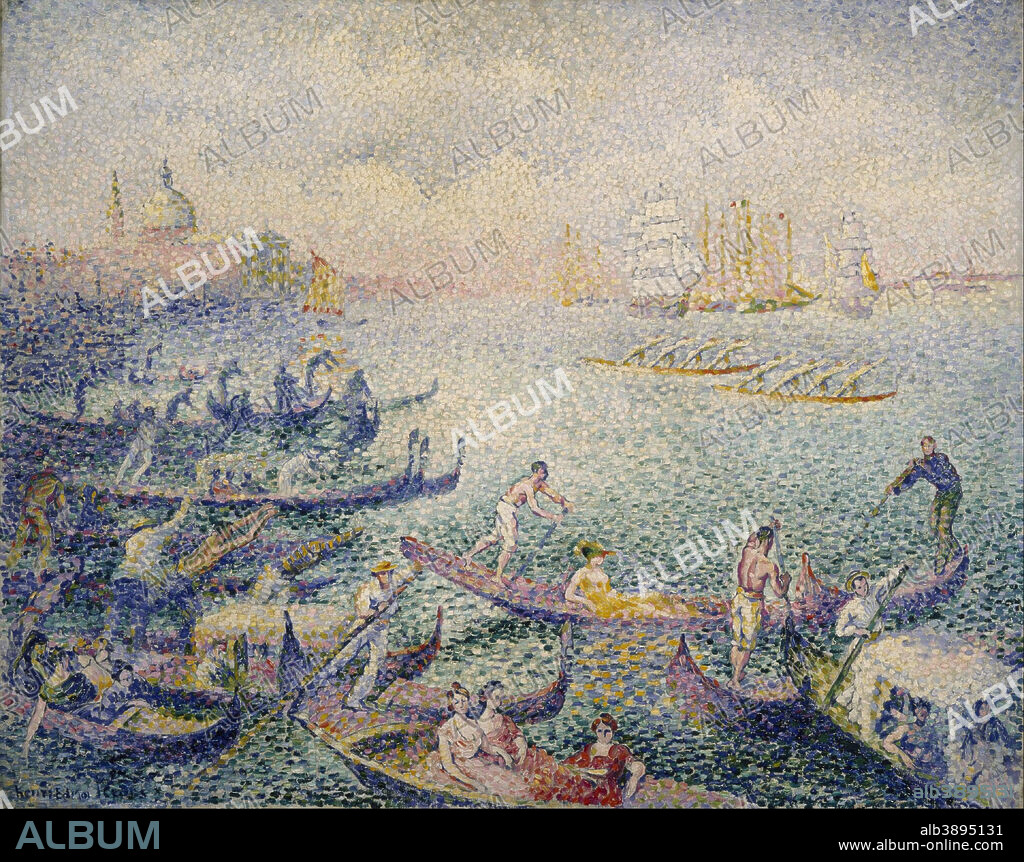This square, multi-colored painting adopts an impressionist style with elements of pointillism. It vividly depicts a bustling water scene set against a serene backdrop. Dominating the lower-left corner and stretching across the bottom of the image, a cluster of gondolas, primarily in bluish-purple with light pink highlights, navigates a large greenish-blue body of water. The gondolas carry women passengers, while men stand on the backs, maneuvering with long poles. Further into the background, larger sailing ships dot the horizon, hinting at the expansive nature of the scene. In the distance to the left, a cityscape resembling Venice emerges softly against a light grayish-blue sky. 

A repetitive watermark reading "ALBUM" in white and blue covers the entire background, with an additional detail along the painting's black bottom border. On the lower left, ALBUM is printed again in blue, and on the lower right, a website, www.album-online.com, appears beside a code, ALB3895131. This combination of vivid colors—blues, yellows, reds, pinks, greens, whites, and grays—and meticulous details captures a lively snapshot of an era gone by, juxtaposed with digital elements pointing to its modern presentation.